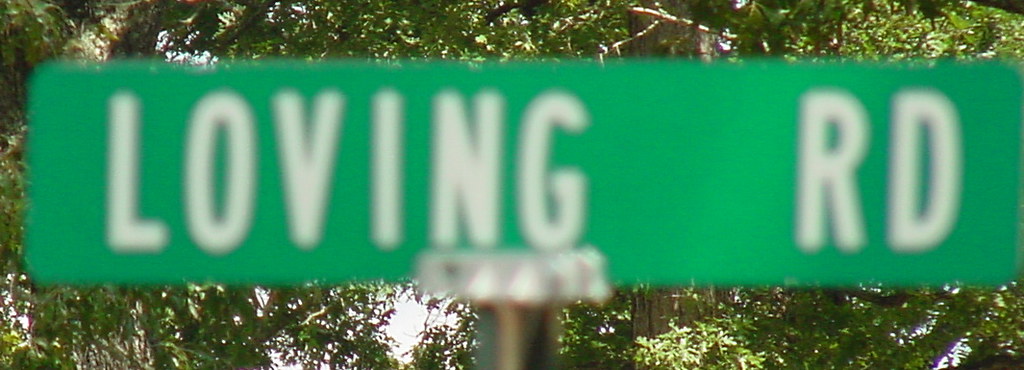The photograph depicts a close-up of a green, rectangular street sign that reads "Loving RD" in white text, mounted on a shiny, dark gray pole partially visible at the bottom. The sign is slightly off-center, extending beyond the right edge of the rectangular frame, while a gap on the left side reveals a peek of greenery. The background showcases a canopy of lush green leaves attached to trees, with a prominent brown and gray tree trunk visible towards the middle right. Although the sign is intended to be the focal point, the image is somewhat blurry, focusing more on the verdant background rather than the street sign in the foreground. The overall scene is illuminated by natural light filtering through the leaves.